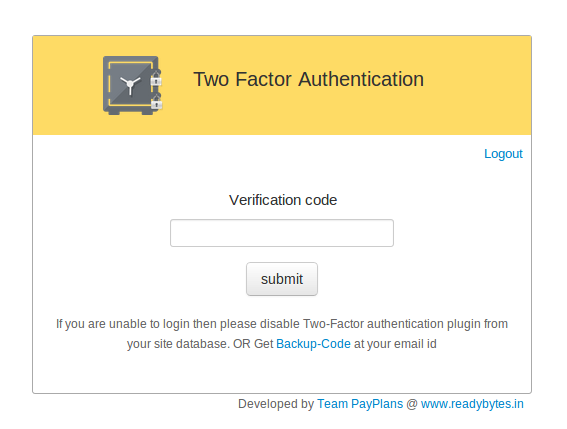This image depicts a two-factor authentication interface. At the top, a black-bordered section with an orange background displays the text "Two-Factor Authentication" in black, accompanied by a gray illustration of a vault with two white lockers and a rotary dial featuring three pins. Beneath this header, the background transitions to white. On the right side, blue text reads "Log Out." Centrally, there's a field labeled "Verification Code" for users to input their code, with a gray "Submit" button below it. Further down, a message in black advises that if users are unable to log in, they should disable the two-factor authentication plugin from their site database or retrieve a backup code sent to their email ID. The term "backup code" is highlighted in blue. Outside the authentication box, at the bottom right, it reads "Developed by Tim Peplens at www.readybyte.in," with both "Tim Peplens" and the URL in blue.